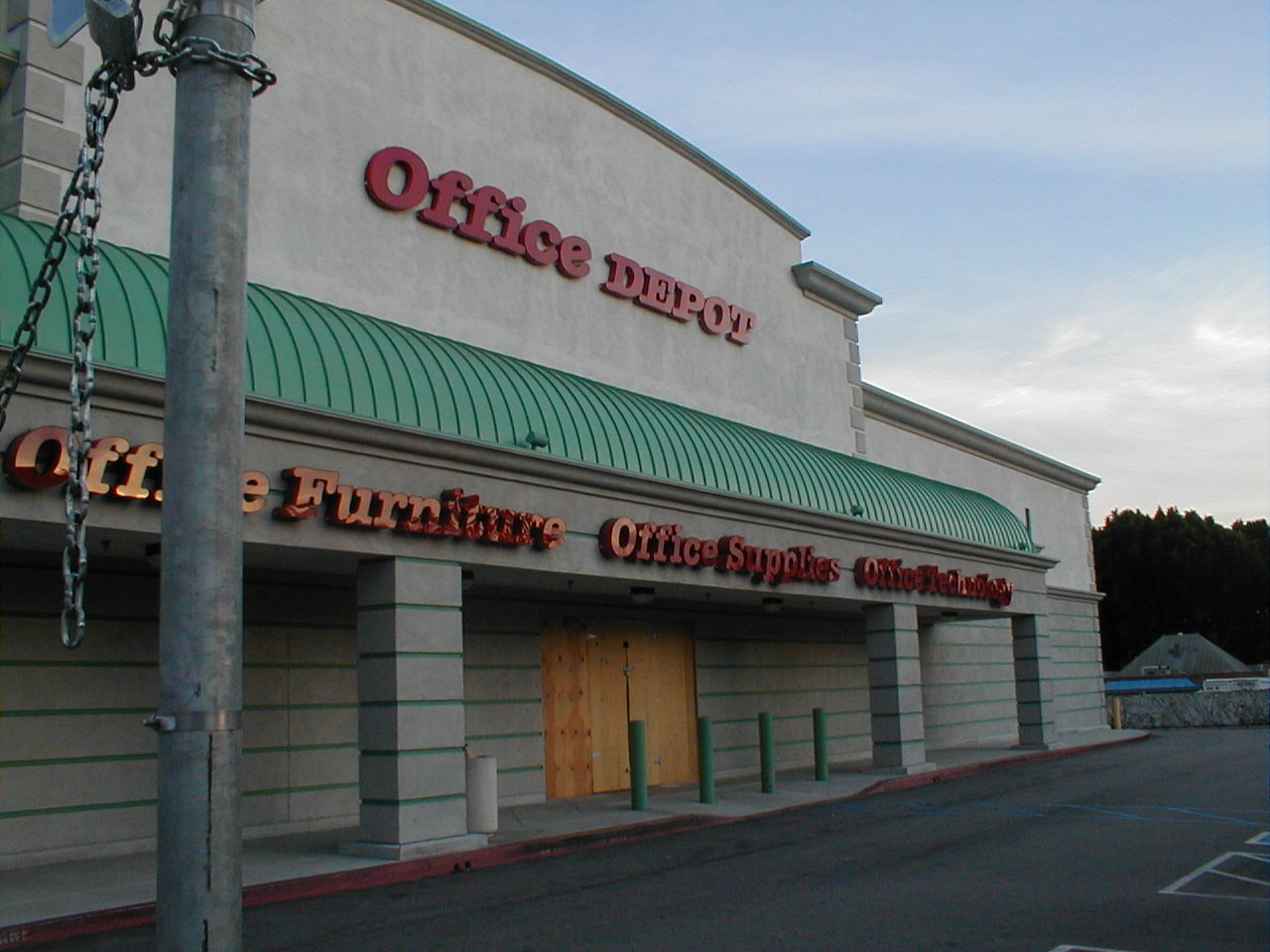The image captures a high-quality photograph of a closed Office Depot building during the late afternoon. The view is from the left side of the main entrance, angled at 45 degrees from the front of the structure. In the left foreground, very close to the camera, stands a grey metal pole with a chain hanging from it. Dominating the main background of the image is the large grey building with green accents, featuring a prominent "Office Depot" sign in red letters at the top. Below the awning, the building displays additional text: "Office Furniture, Office Supplies, and Office Technologies." The sidewalk beneath the awning, lined with a few grey and green pillars, leads up to the now-boarded-up doorway positioned directly at the center of the building. Above, the sky is a mix of blue with some overcast clouds, while some trees can be seen off to the right of the building.